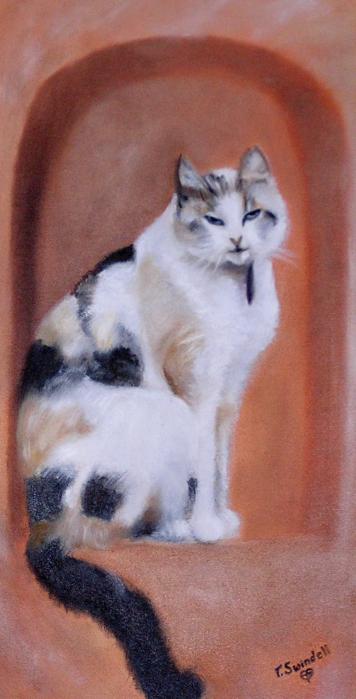This detailed painting depicts a calico cat sitting in a recessed, arch-like shelf built into a wall, resembling a decorative niche or cave. The predominantly white cat, accented with spots of black and orange, has a notably black tail and striped markings on its head and shoulders. The cat’s paws are white, and its slightly closed eyes give it a smug expression as it stares outward. Its whiskers are delicately painted, and it has a pink nose. The background features a reddish-brown, clay-colored wall that complements the cat’s fur. In the bottom right corner of the painting, the artist's signature reads "E. Swindell" with a heart motif underneath.